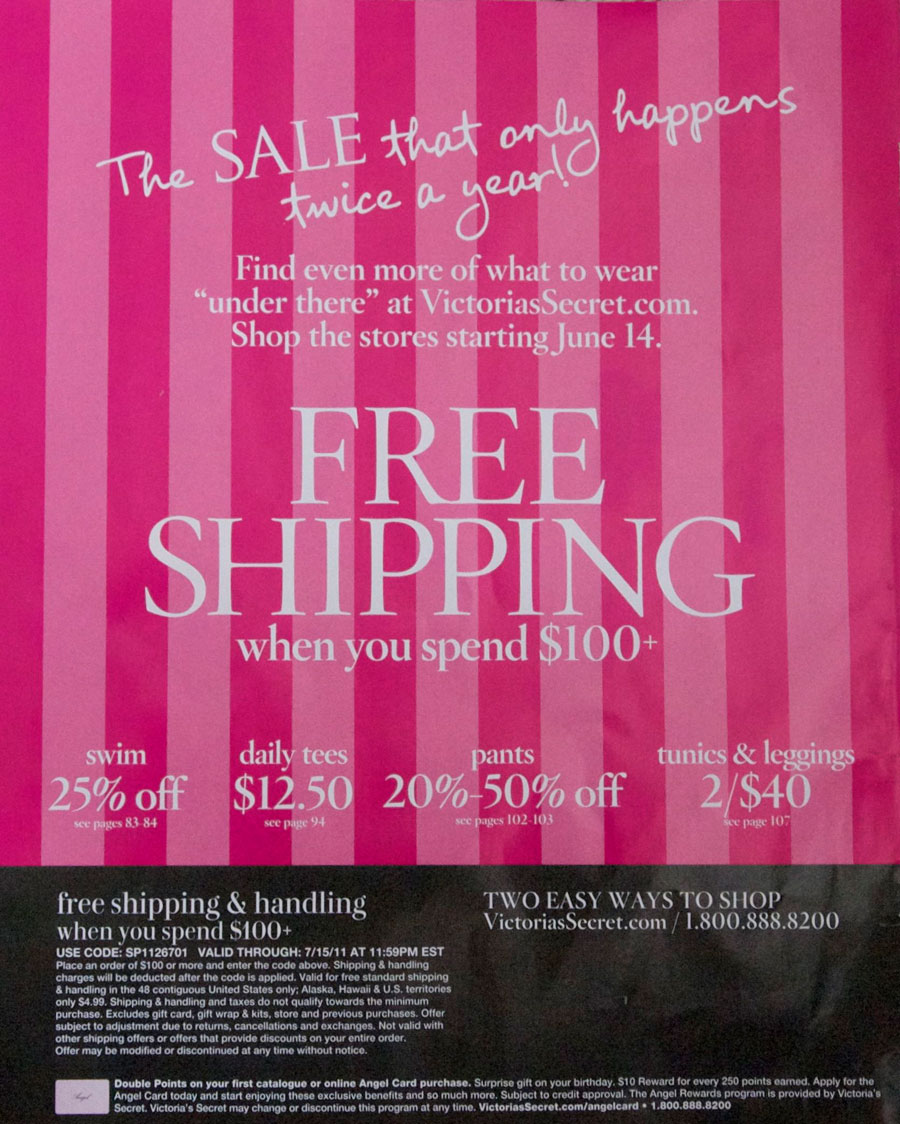The advertisement features bold vertical stripes in shades of red and hot pink, making the white text somewhat difficult to read against the vivid background. At the top, in a stylized, cursive font, it announces "The SALE that only happens twice a year." Below this, it encourages shoppers to "find even more of what to wear under there at victoriassecret.com," and invites them to shop the stores starting June 14th. Prominently in the center, large capitalized text declares "FREE SHIPPING" with the stipulation "WHEN YOU SPEND $100 plus" beneath in smaller font. Various discounts are listed: "SWIM 25% OFF," "DAILY TEES $12.50," "PANTS 20%-50% OFF," and "TUNICS AND LEGGINGS 2 FOR $40." The bottom section of the ad transitions to a black bar with white text detailing the fine print for the free shipping offer, including a required code, its validity period, and terms applicable to the contiguous US states. Additionally, it provides two ways to shop: online at victoriassecret.com and via phone at 1.800.888.8200. The ad is packed with promotional information, despite the challenging readability due to its vibrant design.